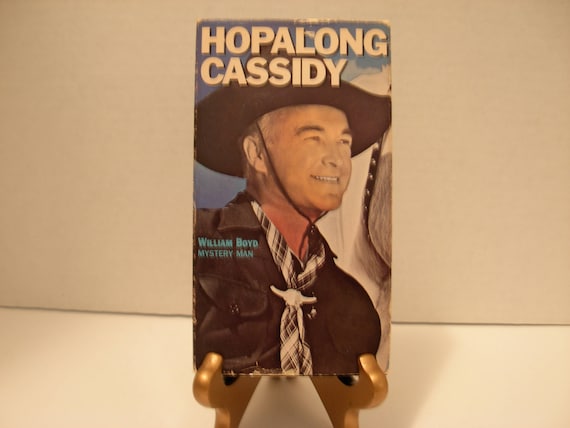The photograph depicts a vintage VHS tape, prominently featuring the title "Hop Along Cassidy" in large white font at the top. The image has a light sepia tone, lending it a nostalgic feel. On the cover, there's a picture of an older cowboy smiling and looking off to the right. He wears a black cowboy hat with a strap and a black cowboy shirt. His neckerchief is patterned in black and white check design and is fastened with a clasp resembling a skull, possibly of an ox. He stands next to a white horse, with only the back of the horse's jaw visible. The VHS tape is placed on a display stand, with an incandescent light casting a warm glow on it, and is set against a white backdrop that appears to be inside a box. The cover also features the text "William Boyd, Mystery Man."